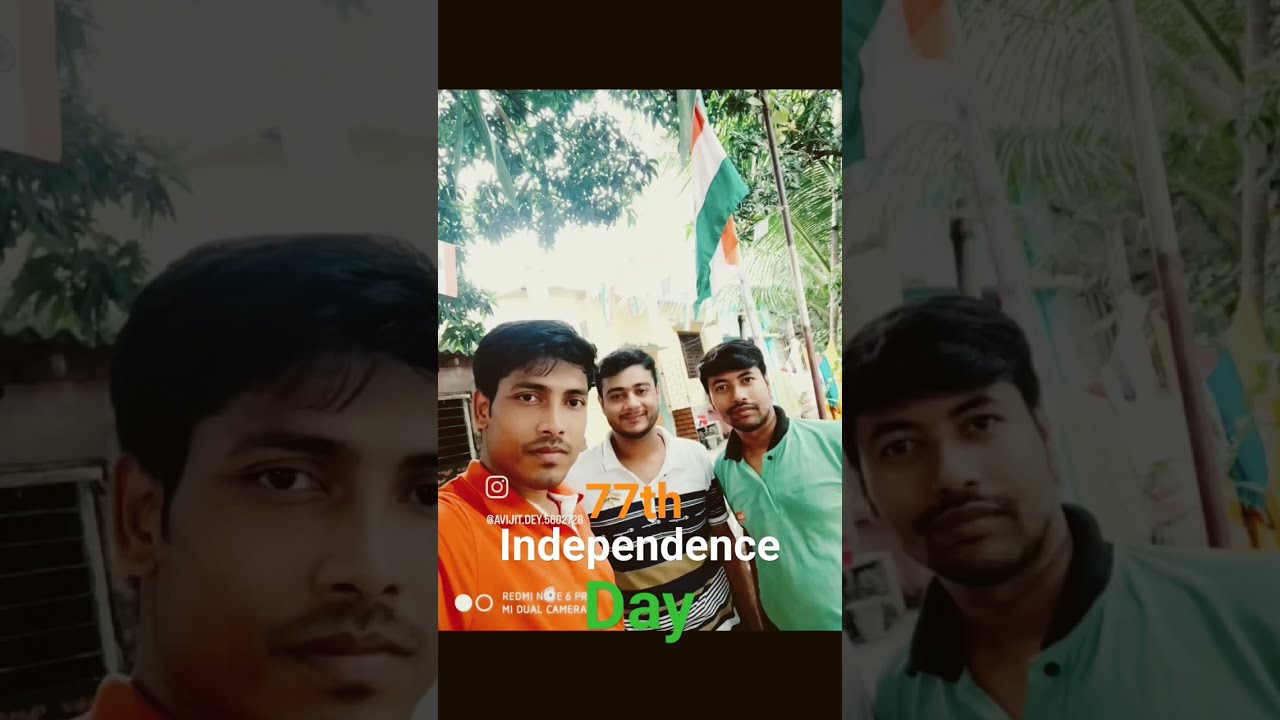The image is composed of three rectangular panels; the side panels have a translucent, darker filter, zoomed-in versions of the central brightened and focused image. The main picture features three young men with black, short-cropped hair, olive skin, and varying types of facial hair ranging from light stubble to more defined mustaches and beards. They appear to be in a tropical outdoor setting, with tree branches and a flagpole in the background, suggesting a natural, sunlit environment. The man on the left, who is taking the selfie, is wearing an orange polo shirt with a white inside collar. The man in the middle is slightly smiling, clad in a white polo shirt with navy blue and beige stripes. The third man, positioned to the far right, gazes seriously into the camera while wearing a seafoam green polo shirt with a dark collar. Above them, a building is visible, though overexposed, and there is an Indian flag on a pole to the right. Below the central image, text reads "77th Independence Day," with the number in orange, "Independence" in white, and "Day" in green. An Instagram icon and social media handles are also visible.